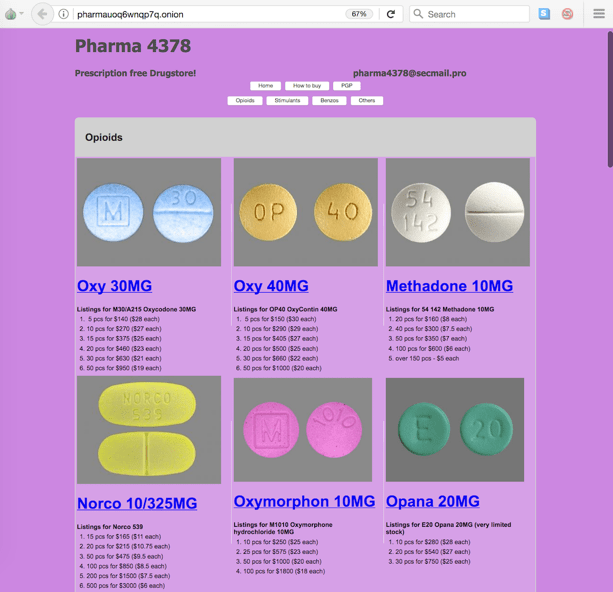A detailed screenshot of a pharmacy website featuring various medications is shown. The URL displayed on the browser is "pharmaq6wnaq7q.onion." The webpage features a purple background with black text, prominently stating "Pharma4378: Prescription-Free Drugstore." Contact information is provided via email at "pharma4378@secmail.pro."

Displayed medications include:

1. **Oxycodone 30 mg**: Illustrated by two small blue pills.
2. **Oxycodone 40 mg**: Signified by yellow pills.
3. **Methadone 10 mg**: Shown as two white pills.
4. **Norco 10/325 mg**: Depicted by yellow pills.
5. **Oxymorphone 10 mg**: Represented by pink pills.
6. **Opana 20 mg**: Marked by green pills.

Each medication is clearly labeled with its name and dosage, highlighting the availability of high-strength prescription drugs without requiring prescriptions.